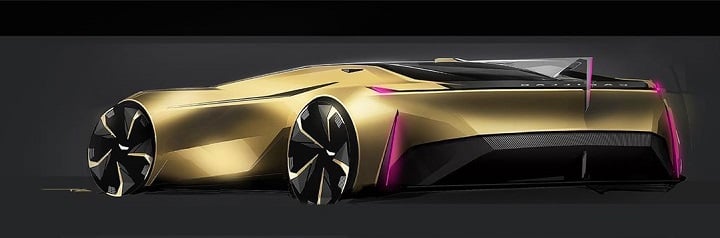The image features a digitally illustrated, low-resolution concept car positioned in a sleek, narrow landscape orientation with a black border at the top. The futuristic car is primarily golden-colored, with a wide and angular yet smooth and aerodynamic shape. The front of the car faces the left side of the image, showcasing large, five-spoked black wheels with gold accents and veined hubs. 

The vehicle has a low design, requiring the driver to sit or lay down to see through the minimal windshield. Decorative purplish lights adorn each side of the front fender, stacked one above the other. The rear of the car features a black diffuser at the bottom of the bumper, a silver and black fin extending from the black roof, and thin cyan-colored taillights. The background is a dark gray, making the car's sleek, golden body stand out prominently.